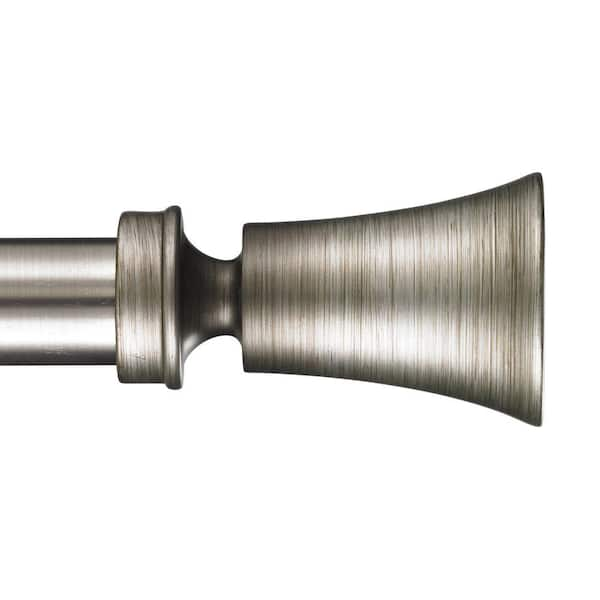The image depicts a sleek and lustrous object, likely a 3D rendering due to its high shine and chrome-like finish. The focus is a metallic, spring-loaded doorstop with a protruding end that suggests flexibility for bouncing up and down. The object is distinctly silver with no other colors, enhancing its polished and reflective appearance. Adding to its complexity, the item resembles a curtain rod's end piece, characterized by brushed stainless steel texture and vertical lines, reminiscent of a sideways bell. The isolated object against a plain backdrop emphasizes its sculptural form and industrial aesthetic.